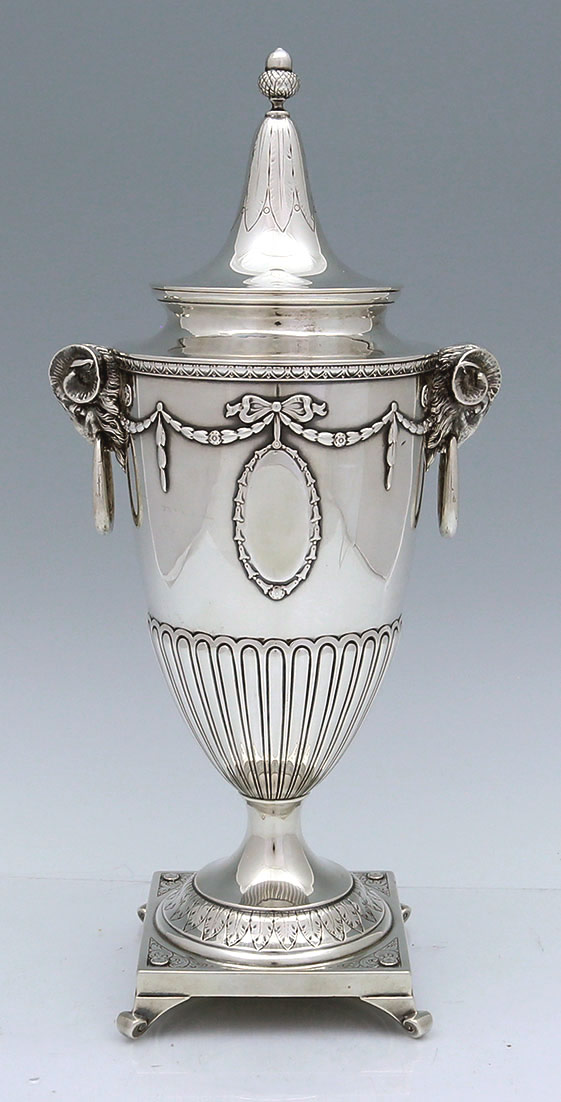The image showcases a large, antique silver trophy with intricate detailing. The trophy is placed on a gray table against a gray background. It features a prominent, covered cup at the top, capped with a metallic, bell-shaped lid that has a small knob or dome with a puffy ball below it. The main cup boasts a design reminiscent of curly flower petals, with handles adorned with confetti-like ring lines converging at a central mirrored or oval medallion. The lower part of the cup has vertical rectangular bar lines that merge at the base, which is supported by a square base with pointed legs. The overall appearance is that of a grand, heavy, and ornate silver trophy, possibly awarded for a significant achievement. The trophy's detailed embellishments, ribbons draping its sides, and its considerable size—estimated to be a couple of feet tall—underscore its impressive and historic nature.